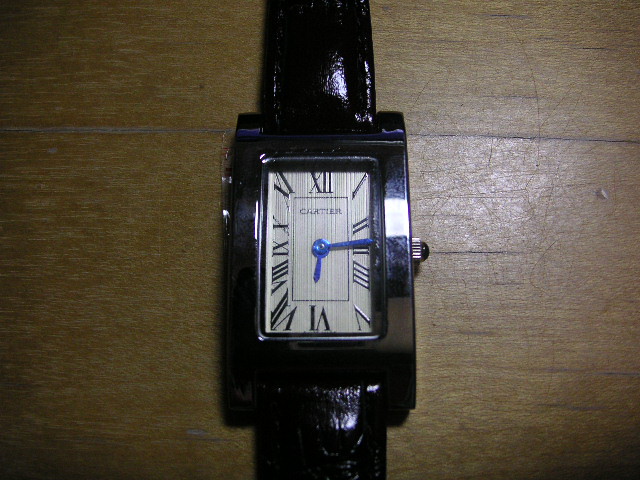This close-up photograph features a rectangular watch with a stainless steel frame, positioned vertically on a well-aged brown wooden table. The watch has a black leather band that appears shiny and thin. The face of the watch is a light tan color, adorned with Roman numerals in black, and blue hands that stand out against the dial. A small dial is situated on the right side of the frame. Although the brand name is difficult to read, it seems to say Cartier. The wooden surface beneath the watch has visible scratches and a horizontal grain pattern, adding character to the composition.